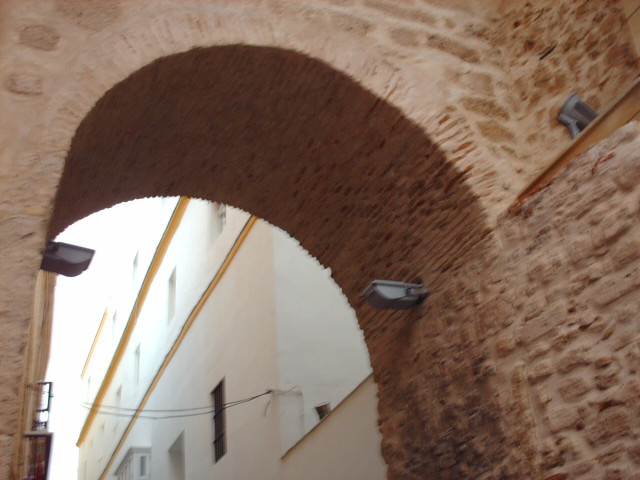The image depicts a picturesque arch-shaped entrance made of brown bricks and cobblestone, situated in an outdoor setting that exudes an aged charm typical of European communities. The structure, with its red and tan bricks, forms a walkable archway whose foundation is a blend of stone and concrete, hinting at its historical construction. Affixed inside the arch are two spotlights, one on each side, likely to illuminate the space at night. Beyond the arch, a white building stands prominently with at least three levels, adorned with numerous windows and trimmed with a yellow or light brown siding. The daytime scene shows natural light flooding the area, with electrical wires stretching from the white building to another structure, encapsulating a harmonious blend of old-world architecture and modern utility.